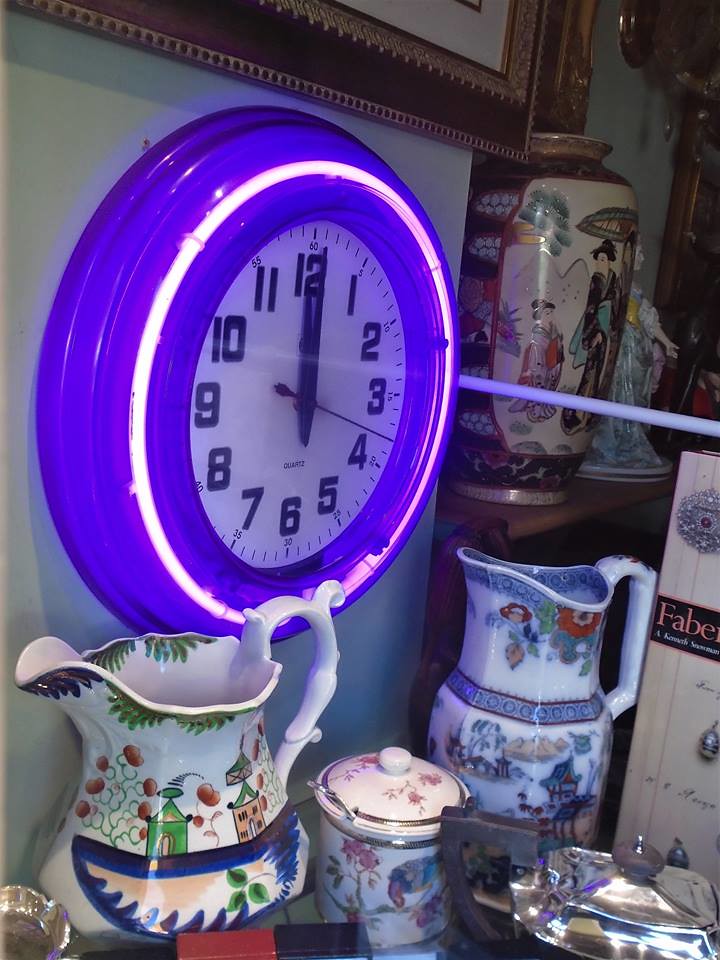The image showcases a vivid, detailed interior of what appears to be an antique shop or a similar setting. At the heart of the image is a clock hanging on the left-hand side of the wall, catching immediate attention with its bright purple casing and surrounding neon ring that emits a glowing white light, further illuminating the purple frame. The clock's face is white, marked with black numbers ranging from 1 to 12, and bordered by minute markers counting by fives up to 60. The black hour and minute hands align at 12, while the red second hand points just before the 4, indicating a time slightly past 12:18. Below the clock, the scene features a collection of vibrant porcelain and china. Numerous intricately decorated vases exhibit colorful illustrations of flowers, plants, and figures in traditional kimonos. Among these items is a tin or steel candy dish and a more distinctive pot with Asian-style patterns of pagodas and flowers. A picture frame, partially out of view, hangs above the clock. In the distance, a shelving unit displays additional vases and a porcelain figure of a woman, completing the rich, eclectic tableau of this quaint setting.